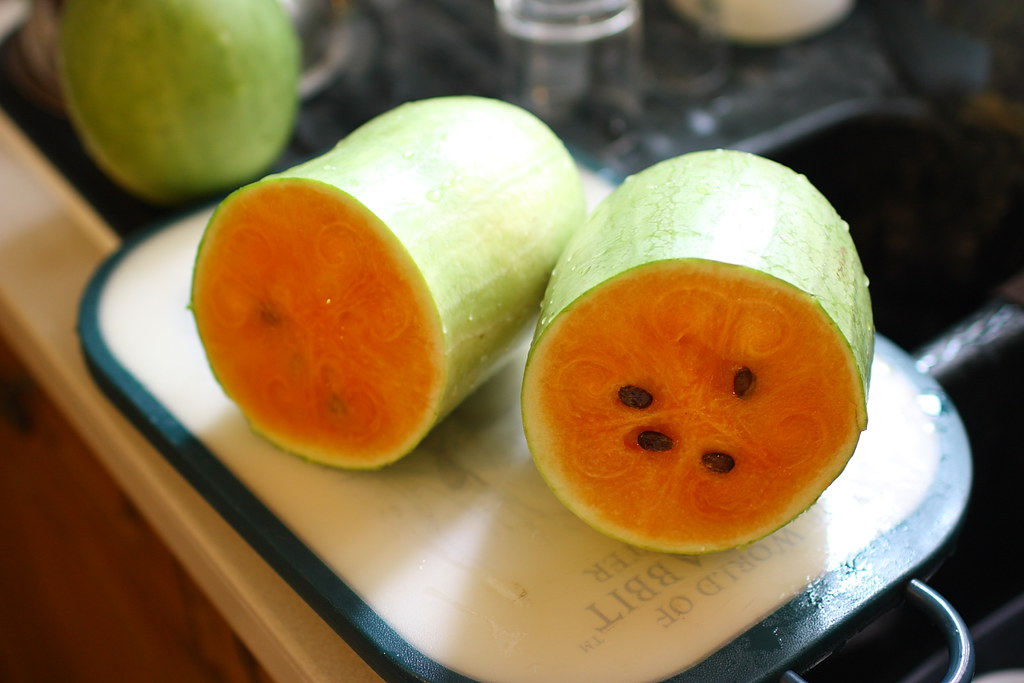The image is a color photograph of a small, tubular-shaped melon, possibly a Sweet Siberian watermelon, which has been sliced crosswise to reveal its pinkish-red inner flesh and large black seeds. The watermelon sits on a white and blue Beatrix Potter-themed cutting board, with a dark blue or black border, positioned above what appears to be a sink. Surrounding the scene are jars and other fruits on the table. In the background, there is another rounder melon and a small coconut. The outer rind of the melon is a pale green with almost no white rind layer. The cutting board and the sliced melon faces are prominently visible, providing a detailed view of the fruit's unique appearance.